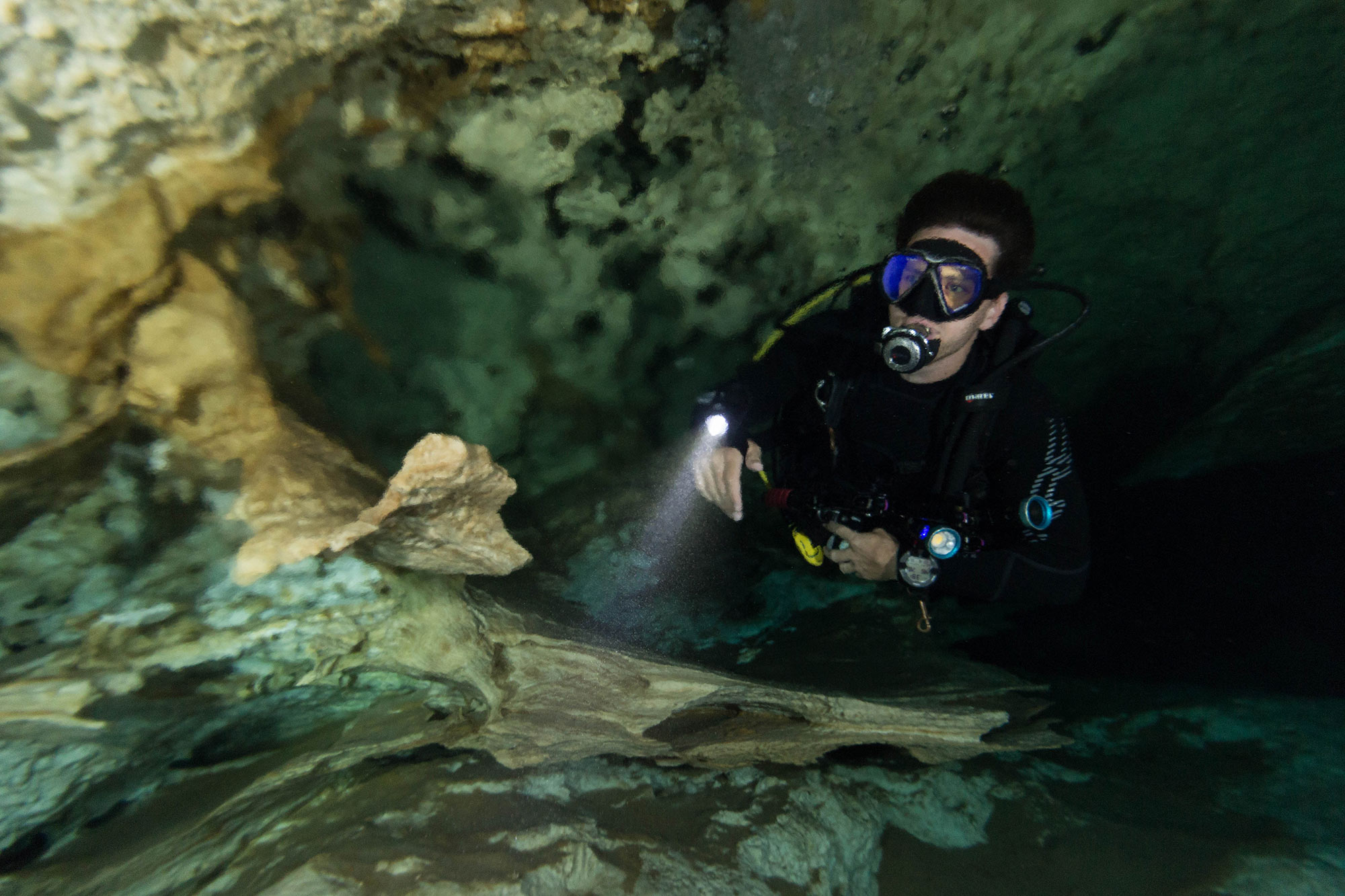In this captivating underwater photograph taken inside a dimly lit cave, a scuba diver in full black wetsuit gear emerges partially from the water, positioned toward the right side of the image and gazing upwards to the left. With blue and black goggles shielding his eyes and a breather securely in his mouth, he navigates the murky cave, utilizing the light from a wrist-mounted flashlight coupled with another handheld light. The cave, adorned with eroded rocky outcrops, showcases a variety of colors—sandy browns, yellows, and shades of grayish-green. The diver, framed by the rugged, jagged edges of the cave walls, reaches towards an indistinct object in the water, adding an element of intrigue to the scene. The dark, foreboding background contrasts sharply with the illuminated rocky foreground, emphasizing the diver's exploration of this mysterious underwater cavern.